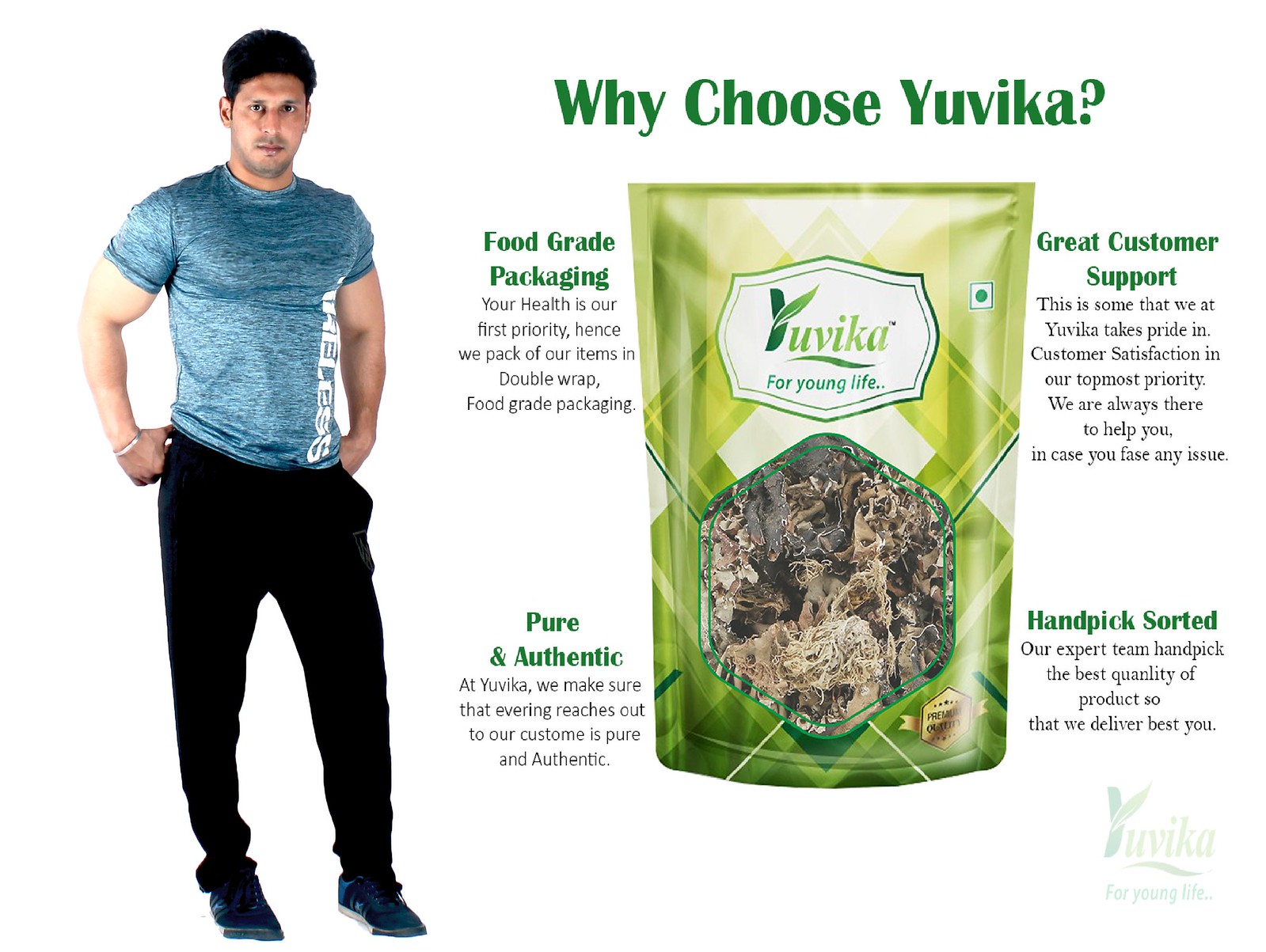The image is a color promotional piece with a white background that seamlessly blends into the screen. It features a muscular man of Caucasian descent with black, slightly fluffy hair, standing on the left-hand side, facing the viewer directly with his mouth closed. He has an oval-shaped face and wears a shiny blue short-sleeved athletic shirt that highlights his built muscles, along with long black pants and blue sneakers. Below the vertical white logo on his shirt, the word "Wellness" appears in white text.

To the right of the man is a green package with the Yuvica logo. The package is partially visible through a six-sided clear window on the front and features a green diamond-shaped checkered pattern. The headline above the package reads "Why Choose Yuvica?" in bold green font. Underneath the headline, several sections of text elaborate on the benefits of the product: "Food Grade Packaging: Your health is our first priority. Hence, we pack all our items in double-wrapped food grade packaging." "Pure and Authentic: At Yuvica, we ensure that everything reaching our customers is pure and authentic." "Great Customer Support: We at Yuvica take pride in exceptional customer service. Customer satisfaction is our top priority, and we are almost always here to help you in case you face any issue." "Handpicked and Sorted: Our expert team handpicks the best quality products to deliver the best you."

In the lower left corner, it says, "Pure and Authentic at Yuvica. We make sure that everything reaches our customer pure and authentic." On the lower right, it boasts, "Handpicked and Sorted: Our expert team handpicks the best quality of products so that we deliver the best for you." The promotional piece combines color and product photography with graphic design elements to create an engaging advertisement.